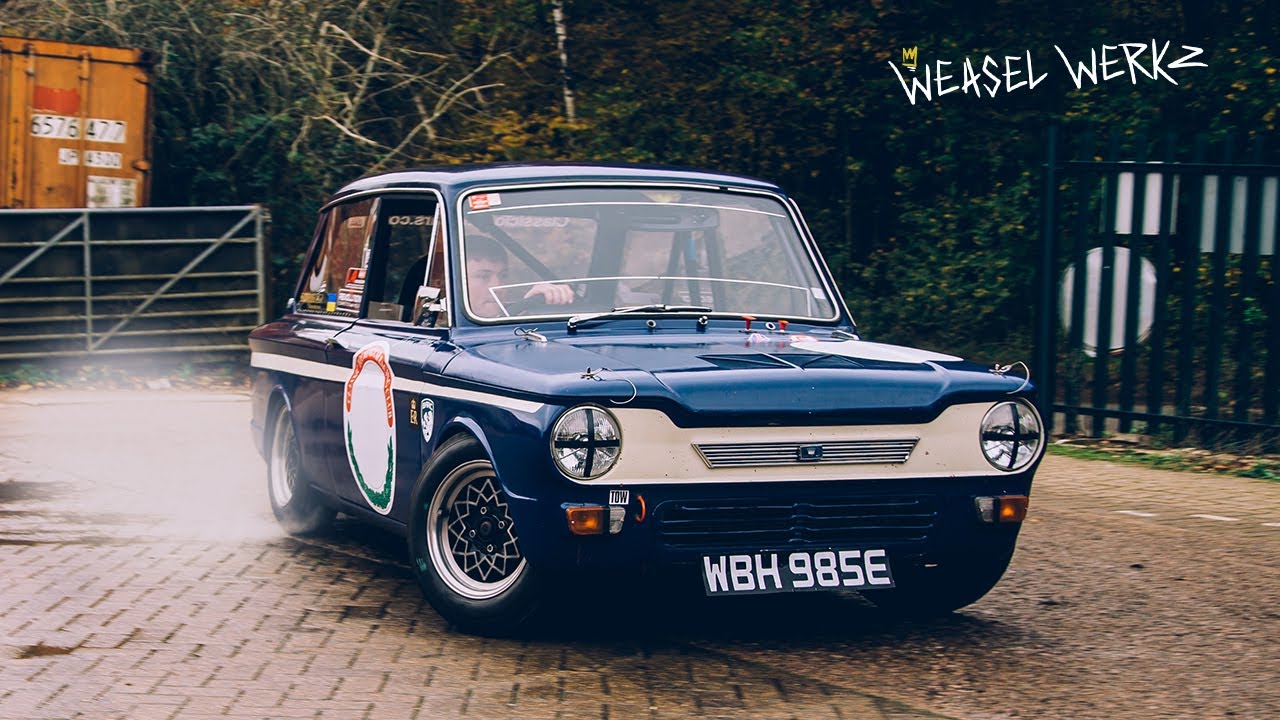The image depicts a compact, royal blue European car driving on a cobblestone road. In the upper right corner, "Weasel Werkz" is prominently displayed in white letters alongside a drawn-on crown. The car, notable for its distinctive appearance, has a license plate reading "WBH-9853," suggesting its European origin. It features round headlights with blue crosses, a white front grille with silver accents, and black wheels with a silver star pattern. 

The driver is seated on the right, with his window down, gripping the steering wheel. The car bears multiple stickers on the rear window and a colorful, bordered white sign on the passenger door, which has an orange and green circle with a red "U." The scene suggests the car might be skidding or burning out, given the visible smoke from the tires.

In the muted background, there is a partial metal fence, dense greenery including trees and bushes, and an orange dumpster marked with the number "6576477." Nearby, a metal gate and a stairwell descending into the shrubbery can also be seen, adding to the outdoor setting which appears to be either morning or afternoon. Overall, the image combines the unique design of the car with a rich, detailed backdrop.